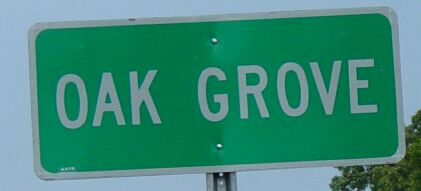A street sign stands outdoors against a backdrop of a clear blue sky, with the edge of a tree visible in the bottom left corner. The sign is mounted on a silver metal pole, which is partially visible. The sign itself is green with "Oak" written in large white letters, and "GROVE" displayed in equally bold white capital letters beneath it. The sign is affixed to the pole with two silver screws. The green background of the sign is accented by a white border that complements the white text. The scene captures the simplicity of the street sign against the natural elements of sky and foliage.